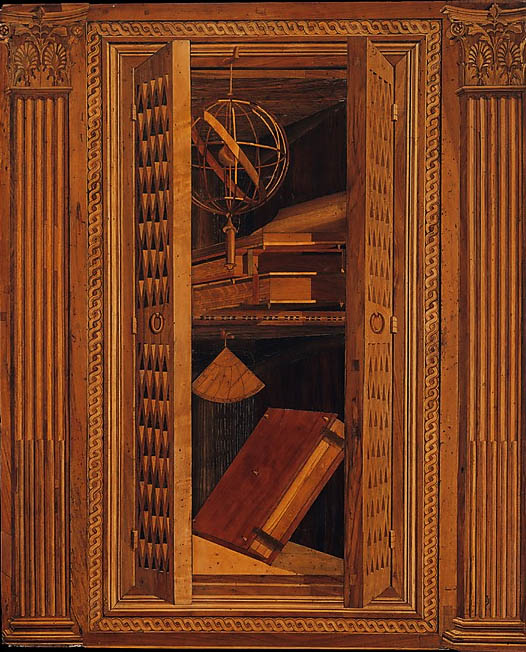This painting is a detailed depiction of an elegant wooden cabinet, captured in a rectangular portrait orientation. The large cabinet is adorned with ornate features on either side, drawing attention to its intricate craftsmanship. The cabinet doors are open, revealing two shelves within. The bottom shelf holds a reddish-brown book, which is notably tilted upwards and to the right. Meanwhile, the top shelf is home to a globe-like object suspended from the top of the cabinet, accompanied by several neatly stacked books. Additionally, the bottom shelf presents a triangular object hanging down from the top shelf, enhancing the cabinet's visual complexity. The entire cabinetry is rendered in a light brown wood, showcasing its fine texture and rich tones.